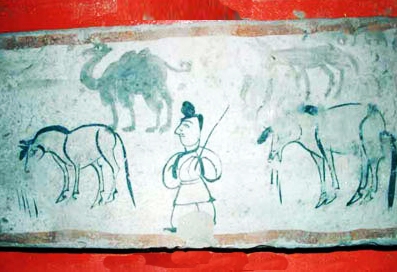The image features detailed artwork designed to mimic ancient cave drawings, set against a stark bright red background. The primary piece appears to be a digitized version, possibly on a silvery or grayish material with elements suggesting a stone surface. Dominating the center of the artwork is a rudimentary human figure, identifiable by a distinctive bun hairstyle and wielding a stick or sword. Surrounding this central figure are four animals depicted in a simplistic, archaic style. On the left side is a line drawing of a horse, while above it sits a more filled-in drawing of a camel. To the right of the man is an unclear animal with multiple legs, and below it, in the bottom right corner, is another horse bending over, seemingly to graze. The artwork is bordered at the top and bottom by brown lines, enhancing its ancient, cave painting aesthetic.